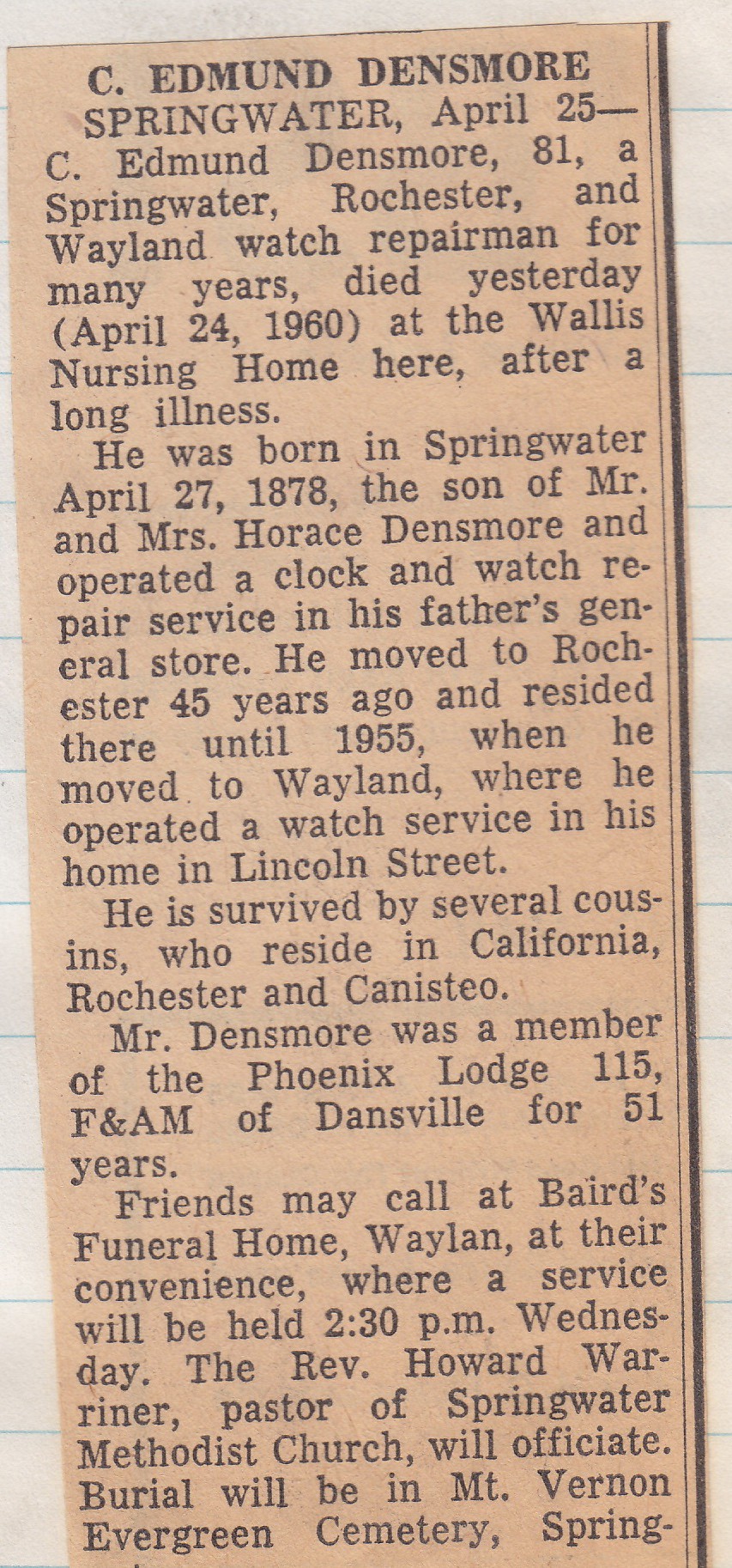The image is a photograph of an aged newspaper obituary laid on lined paper, with visible red, blue, and white stripes. The clipping, in a light orange hue with black text, details the life and death of C. Edmund Densmore. The headline states his name, "C. Edmund Densmore," and the cities associated with him: Springwater, Rochester, and Wayland. The article reports that Densmore, 81, a long-time watch repairman, died on April 24, 1960, at Wallace Nursing Home after a prolonged illness. Born on April 27, 1878, in Springwater to Mr. and Mrs. Horace Densmore, he initially operated a clock and watch repair service in his father's general store. He moved to Rochester 45 years ago and lived there until 1955 when he then relocated to Wayland and continued his watch repair work from his home on Lincoln Street. Survived by several cousins who reside in California, Rochester, and Canesso, Densmore was a dedicated member of Phoenix Lodge 115F and AM of Dansville for 51 years. Friends are invited to call at Brad's Funeral Home in Wayland, where a service will be held at 2:30 p.m. on Wednesday, officiated by Reverend Howard Warriner of Springwater Methodist Church. Burial will take place at Mount Vernon Evergreen Cemetery.